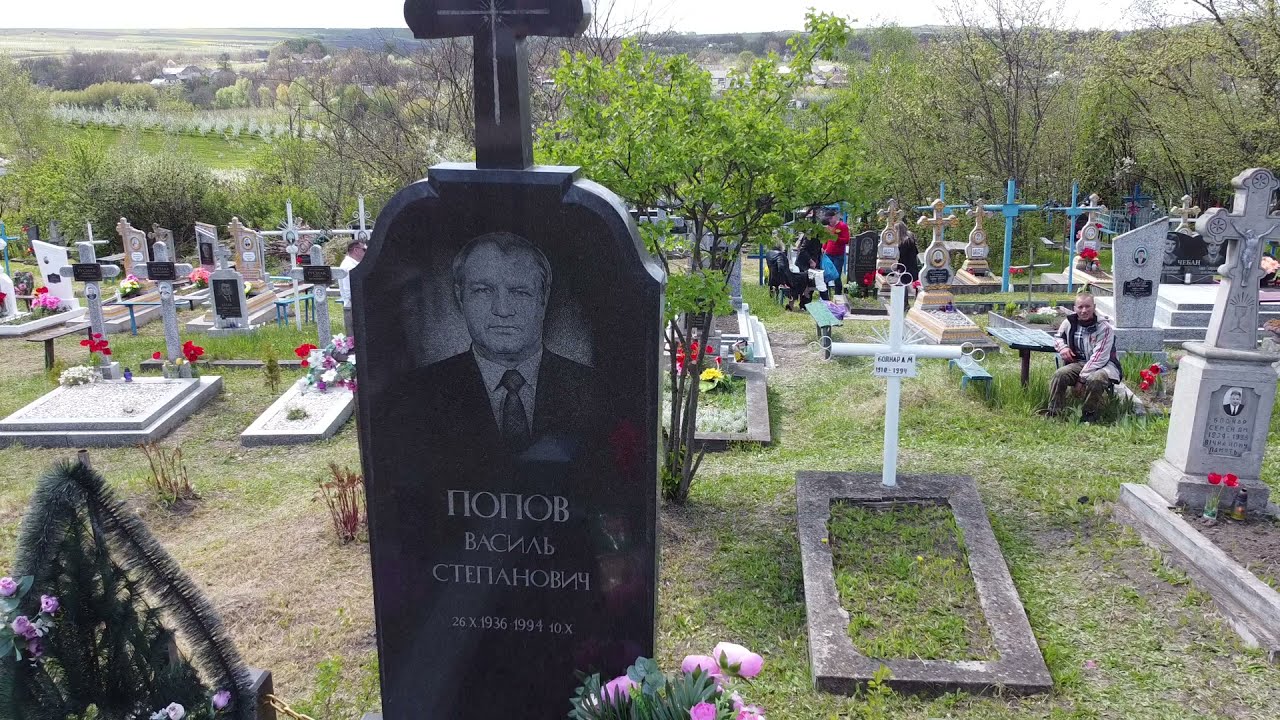The image captures a tranquil cemetery filled with numerous headstones set against a backdrop of patchy grass and numerous trees. Dominating the scene is a large, distinct, black tombstone situated slightly off-center to the left. This headstone stands out among the more common gray concrete tombstones due to its height and color. Engraved on it, in Russian, are the details of an individual who lived from October 26, 1936, to October 1994. Above the Russian inscription is a photograph etched into the stone depicting an elderly man with an "M"-shaped white hairline, dressed formally in a black suit and bow tie.

In the background, additional headstones with crosses and flowers are visible, indicative of a well-visited resting place. Among the visitors, a notable figure is a man sitting on a blue bench on the right side of the image. This man, who bears a striking resemblance to a younger version of the man depicted on the headstone, is dressed in a long-sleeved pink checkered shirt and green pants, and is looking directly at the camera. The serene atmosphere is accentuated by the presence of trees and a glimpse of an urban area further in the distance.